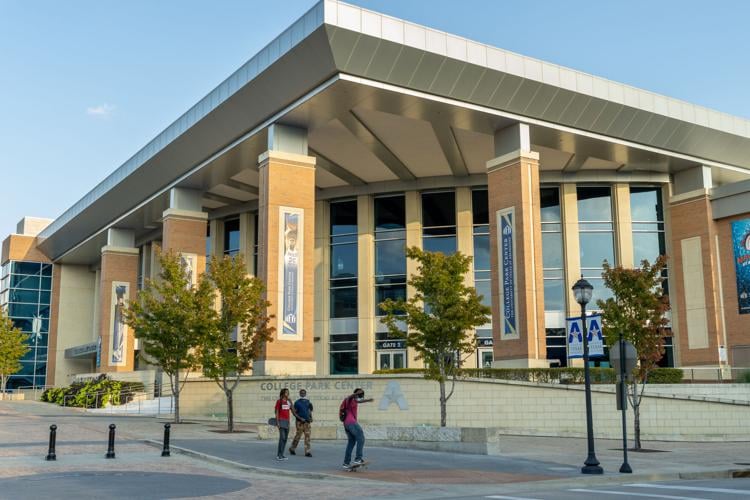The image showcases a modern university building identified as College Park Center, distinguished by its large glass windows and design akin to an auditorium or performance hall. The front of the building features a significant overhang supported by block-shaped pillars, some of which display banners or signs. Set back from the main structure, the entryway opens to a spacious area, hinting at a second floor ideal for congregation and observation, characterized by its flat roof extending to a point at the top left.

In front of the building, amidst leafy trees approximately 20 feet tall and some nearby bushes on the left, three individuals can be seen. One, wearing a red top, holds a skateboard. Another individual, donning a red top, gray pants, and a backpack, is approaching the street on a skateboard. The third person, dressed in a blue shirt and camouflage pants, stands nearby. The scene presents a dynamic yet tranquil academic environment, highlighted by the stone wall bearing the College Park Center name and supported by the visual presence of the orange rectangular columns.